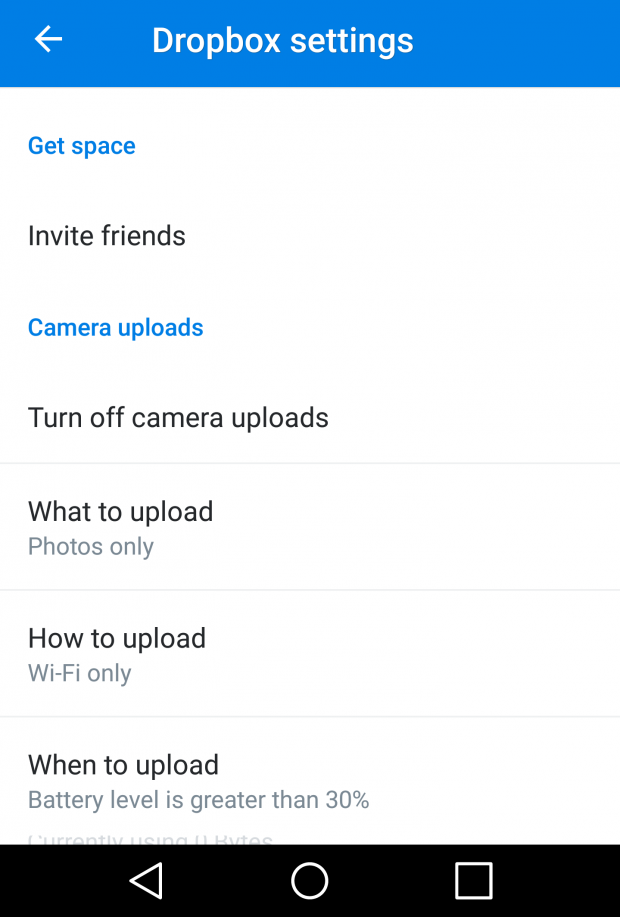This detailed caption describes a screenshot taken from an Android smartphone displaying the Dropbox settings menu. 

---

The screenshot, likely taken from an Android smartphone, showcases the Dropbox settings menu. At the top, there is a blue header bar containing a white left-facing back arrow and the text "Dropbox settings" in white. Below this header, various options are listed in both blue and black text.

1. "Get space" is displayed in blue text.
2. "Invite friends" follows in black text.
3. "Camera uploads" is seen in blue text.
4. "Turn off camera uploads" is in black text.

A faint gray line separates these options from the next section. Under "What to upload," the option "Photos only" is shown in gray text. Another faint gray line leads to "How to upload," with "Wi-Fi only" listed in gray text underneath. 

Yet another faint gray line directs to the "When to upload" section, which specifies "Battery level is greater than 30%" in gray text. Partially visible text beneath this reads "Currently using zero bytes," indicating there are more settings cut off from view.

At the bottom of the screenshot, the typical Android navigation bar is present, featuring a triangle pointing backward (back button) on the left, a circle in the middle (home button), and a square on the right (overview button). The screenshot provides a detailed view of the Dropbox settings related to upload preferences and conditions.